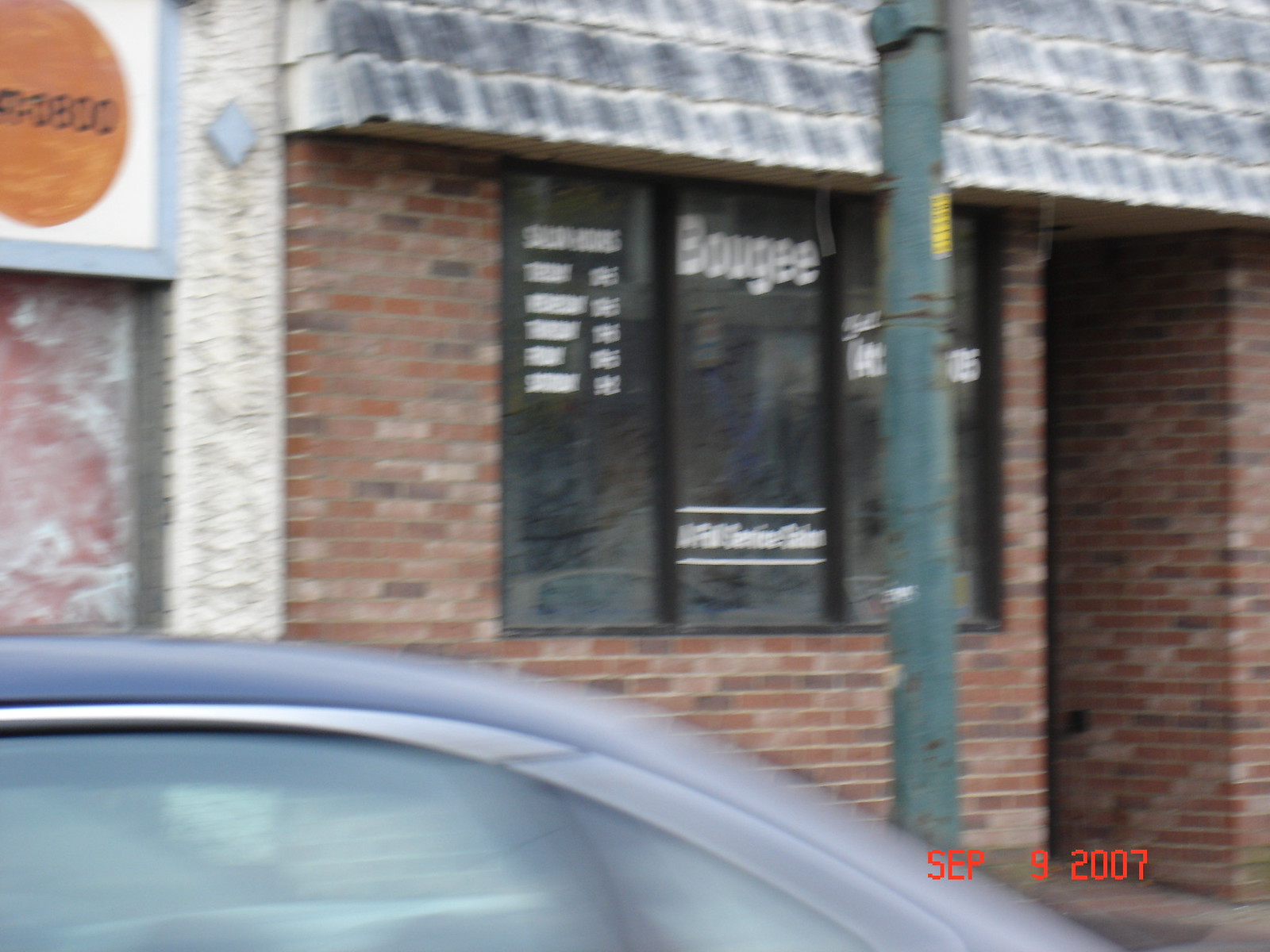This photograph, dated September 9, 2007, captures the exterior of a storefront on an overcast day. Situated in a predominantly red brick building, the storefront features a trio of large windows framed by black supports. The central window prominently displays the word "Bougie" (B-O-U-G-E-E) in white letters, while the other windows feature indistinguishable white text, with the rightmost obscured by a silver metal pole. The upper portion of the photo reveals a weathered, shingle-like valance appearing light gray from exposure, and a building edge with a goldish circle inset containing partially legible black text ending in "800". Beneath, a dirt-darkened stone wall transitions into the red brick façade. A gray stone pillar is visible near the upper left, adding to the rustic urban aesthetic. In the lower part of the image, the roof and back window of a dark blue car are visible, hinting at either parking or movement along the sidewalk. The photograph's timestamp, printed in red text, is located in the bottom right corner.